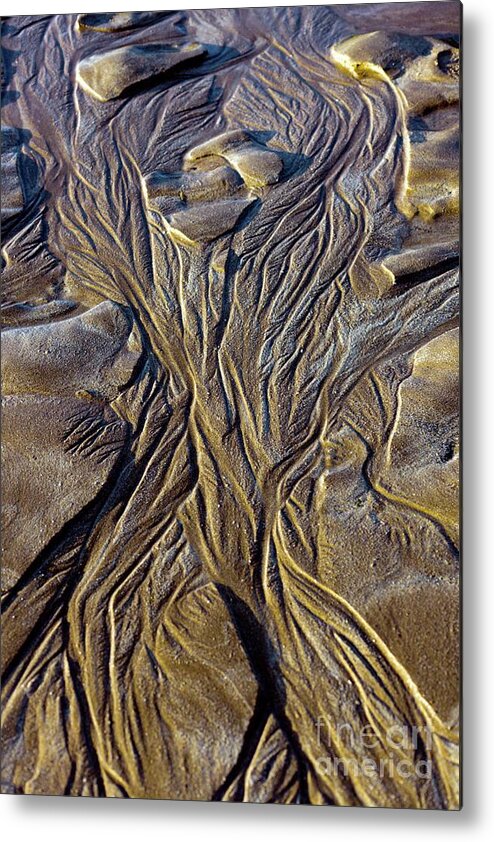The image depicts a detailed, textured art piece that mesmerizes with its complexity. It features a series of intricate rivulets and little valleys carved into a dark brown to golden-brown, sandy or clay-like surface, possibly resembling an area shaped by water erosion in a desert landscape. The surface appears 3D, with elevations and depressions creating a dynamic, organic flow across the scene, enhanced by the natural lighting that highlights its etched details. The colors transition from greenish-beige at the bottom to silvery hues towards the top, adding depth to the composition. Soft, weathered rocks are visible near the top, further contributing to the naturalistic effect. The artwork is not flat; it’s framed, suggesting a higher level of craftsmanship and presentation. In the bottom right corner, the faint but discernible text "Fine Art America" confirms its origin, with the letters in a light gray that blend subtly into the image. The overall impression is of a meticulously created piece that captures the essence of natural landscapes through artistic interpretation.